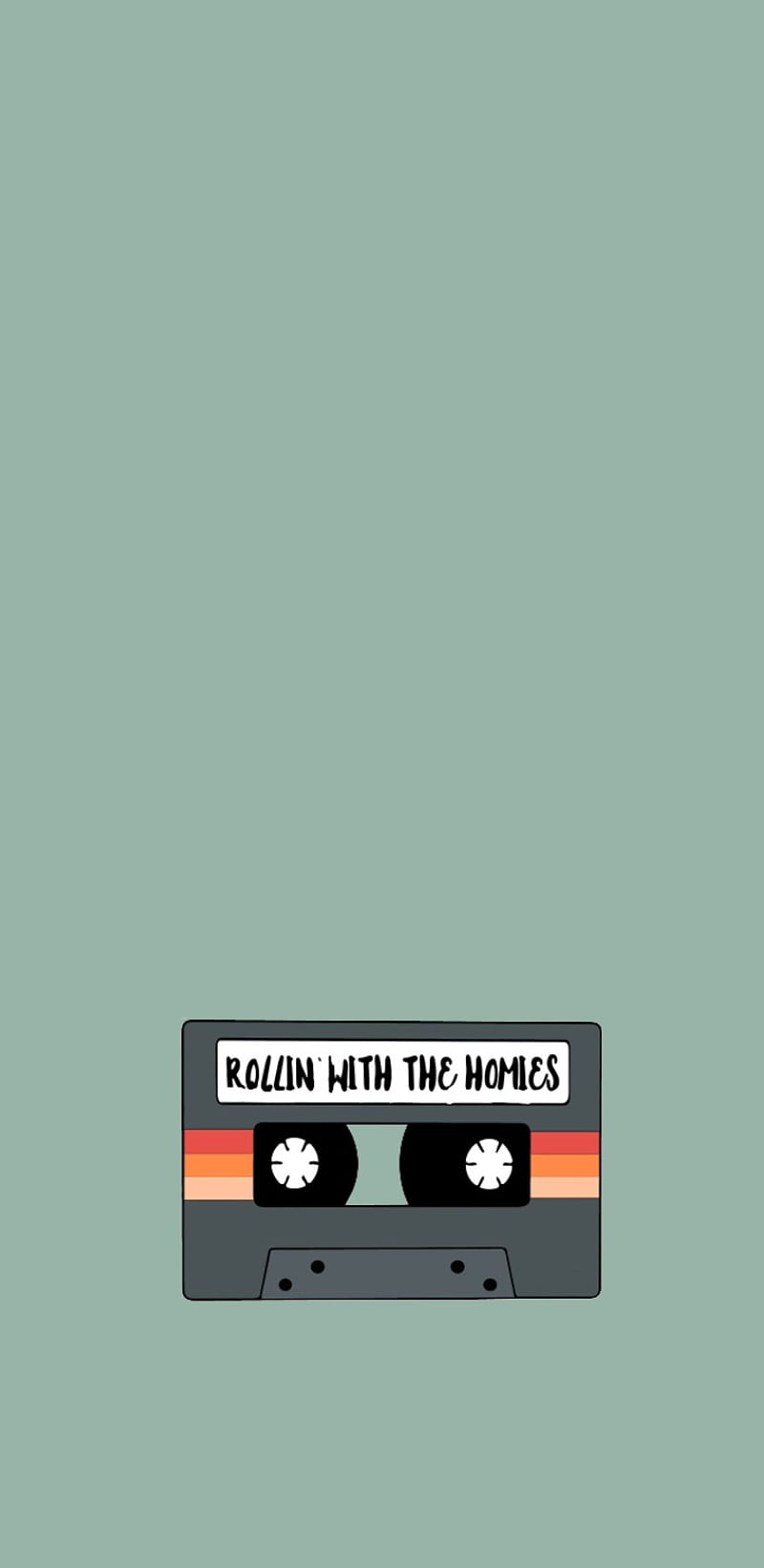The image showcases a moderately small, cartoonish drawing of a gray cassette tape with a handwritten label reading, "Rolling with the Homies." The tape features two white reels, with more black tape on the right reel, indicating it has been played about halfway through. It has a red, orange, and yellow stripe design stretching horizontally across the middle. The cassette is set against a grayish-teal background, positioned toward the bottom third of the image.